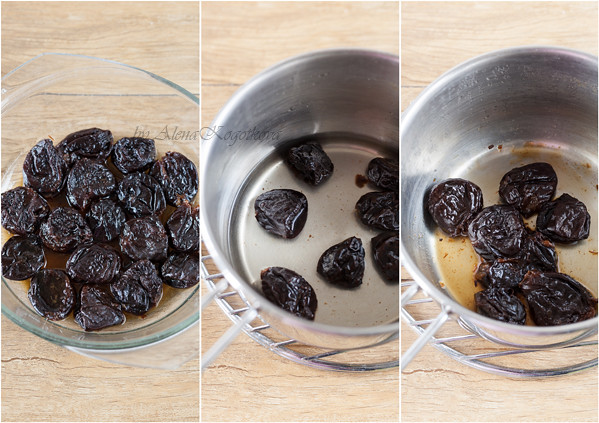This image, taken from above against a light oak wood background, showcases what appears to be the stages of preparing or cooking dates. The photo is divided into three vertical columns. The leftmost column features a glass bowl filled with dark, wrinkled dates submerged in a brownish sauce. In the middle column, the dates are partially submerged in a stainless steel pot, which sits on a metal wire stand. These dates appear to be in water and not yet cooked. The rightmost column repeats the image of the stainless steel pot, but this time the dates are more thoroughly cooked, as indicated by the increased amount of brown sauce at the bottom. A tiny, illegible watermark is present on the image.